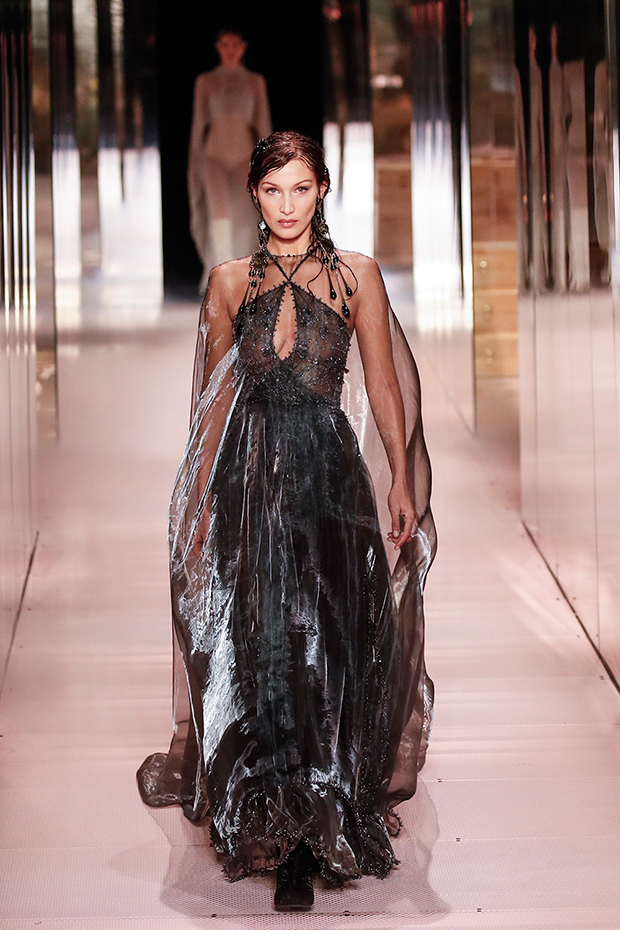The photograph captures Bella Hadid confidently striding down a fashion runway in the spotlight. She is clad in an intricate floor-length black gown, featuring a sheer, lacy fabric adorned with a reflective, metallic sheen. The dress includes a cutout around the chest and a flowing, sheer black veil enveloping her figure, adding to the ethereal quality of her ensemble. A notable detail is the unique headdress: a striking black piece adorned with beads that cascade down her shoulders, emphasizing her sculpted cheekbones and elegant demeanor. Her partially down, partially pulled-back brown hair complements her look, with bangs swooped to the right side of her face. Black shoes peek out from beneath her dress as she proceeds toward the camera, her eyes fixed straight ahead. Behind her, a second model dressed in a similar, sheer white dress appears ready to take her turn on the pristine, white runway, which is accented by mirrors flanking either side and wooden shelving interspersed along the mirrored walls. The sharp stage lighting enhances the reflective details, creating an almost dreamlike ambience.